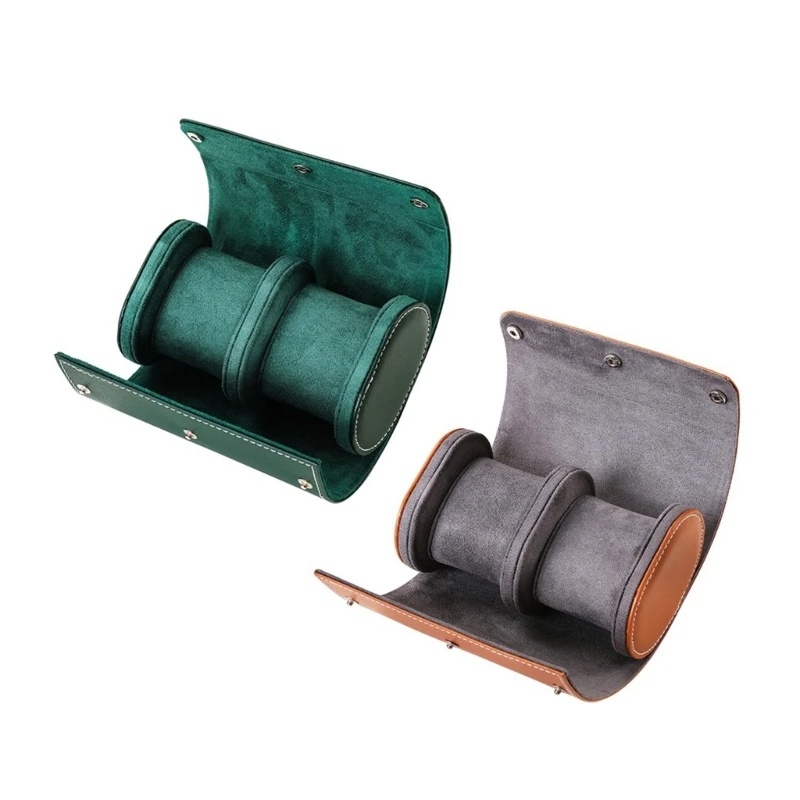The image depicts two leather watch cases, both designed to protect timepieces or bracelets. Each case is shaped like a tubular container, lined with felt and divided in the center by a thick leather ring. At either end of the tube, there are similar thick leather rings which help maintain the shape and facilitate wrapping watches securely around the interior. An outer layer of leather wraps around the tube and is secured by three buttons to ensure the items inside do not get scratched.

The watch case on the left is entirely sea green, with matching green leather on the outside and green felt on the inside. The watch case on the right, however, features a combination of colors: it has gray felt inside and tan leather on the outside. Both cases are detailed with oval leather circles at their ends—black on the green case and orange on the tan and gray case. Despite their differing colors, the structures of the two cases are identical. No watches or bracelets are currently placed inside either case. The leather of both cases shows a well-crafted, slightly indented U-shape, hinting at the soft material’s flexibility and quality.